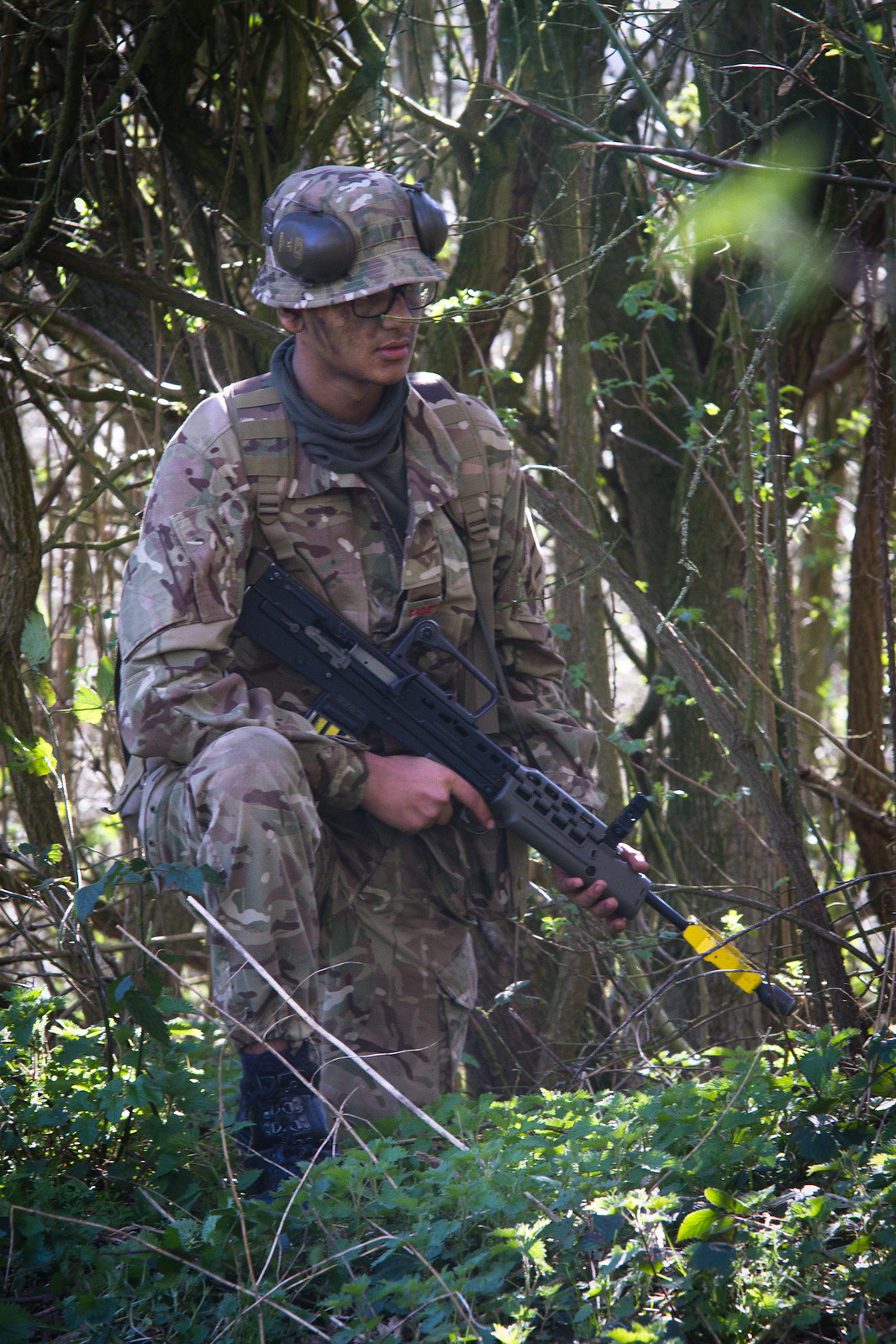The image depicts a young man with medium skin tone and eyeglasses, fully clad in camouflage military attire, including a jacket, long pants, and black boots. He also has a camouflaged hat with earmuffs attached to it, though the earmuffs are not covering his ears. His face is painted in camouflage colors. The man is crouching in a wooded area, surrounded by trees, grass, and other vegetation. He appears focused and concentrated, holding a large, well-maintained rifle. One of his hands grips the rifle while the other is on the trigger, and the end of the rifle is marked with something yellow. It is a sunny day, and there is a sense of alertness and readiness in his posture. He also has a scarf and a backpack, suggesting he is equipped for outdoor activity. The vertical rectangle photograph captures a detailed and immersive scene in the forest, highlighting both his military gear and the lush surroundings.